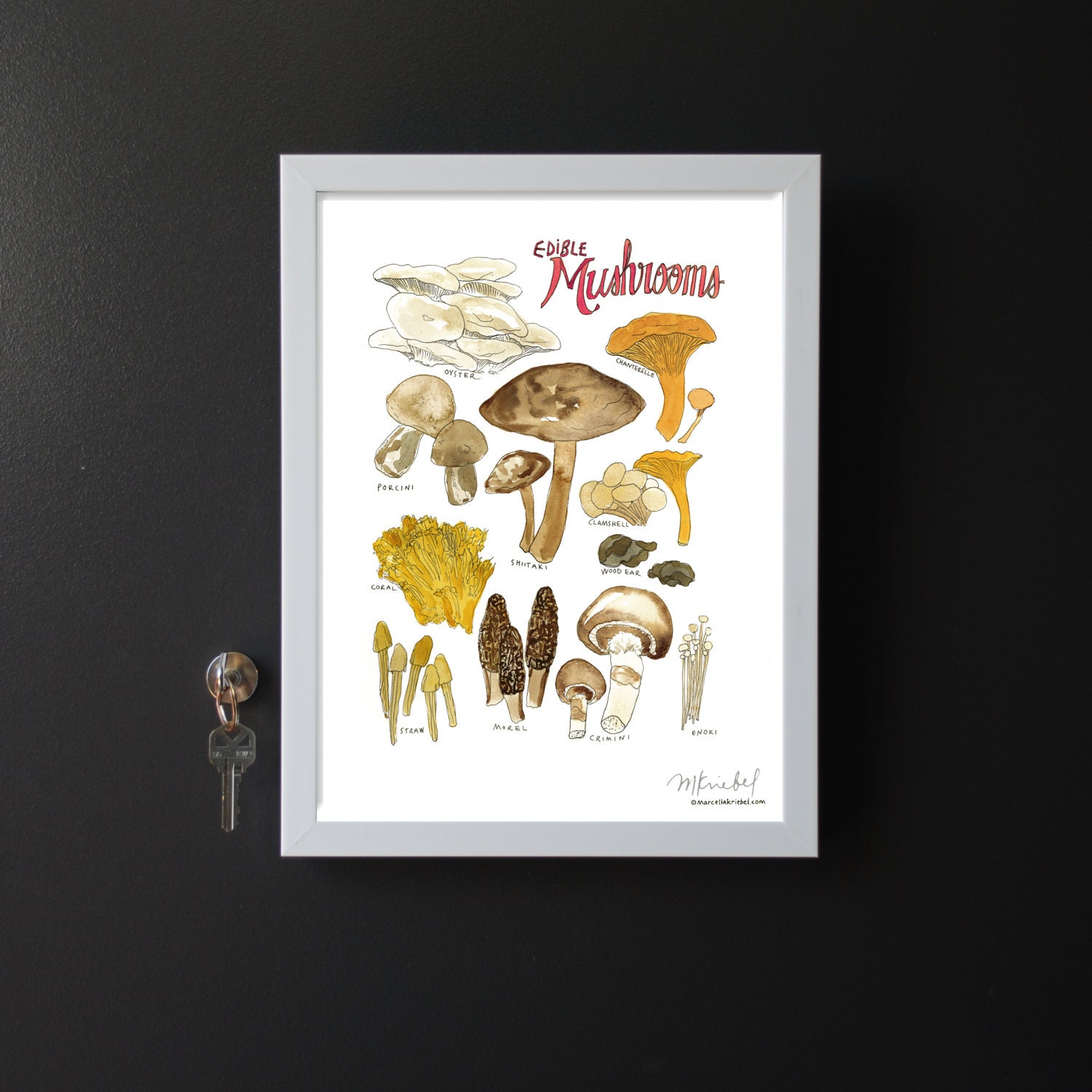The framed illustration titled "Edible Mushrooms" features detailed pen and ink drawings of various mushrooms such as oyster, chanterelles, morels, porcini, shiitake, clamshell, wood ear, cremini, nori, and coral, all rendered in watercolor. The mushrooms are labeled with their names, although the text is too small to read clearly in the image. The artist's name is inscribed in the bottom right corner of the artwork, which is set against a black wall and enclosed in a gray 8 by 10 frame. Adjacent to the framed illustration is a single house key, likely a Kwikset style, hanging on what appears to be a magnetic hook. The key adds an unusual element to the scene, enhancing its domestic setting.